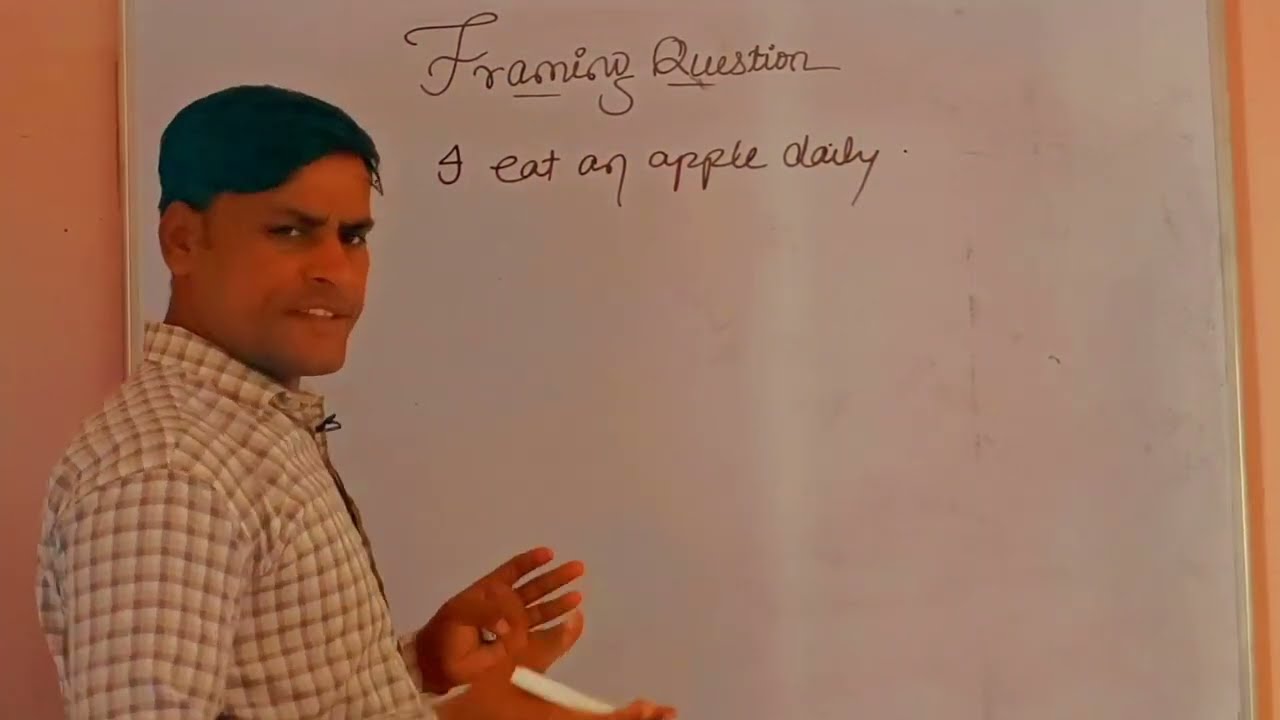In this detailed color photograph, a dark-skinned male instructor, who has dark hair and dark eyes, is captured standing in a classroom in front of a whiteboard. He is positioned slightly to the left side of the image, gesturing with his hands as if speaking to his class. The instructor is dressed in a plaid shirt featuring shades of beige, brown, and white. In his right hand, he holds a white marker, while his left hand, holding what appears to be a marker cap or piece of chalk, is extended forward. 

On the whiteboard behind him, written in black text, are the words "Framing Question" followed by "I eat an apple daily." The background of the scene reveals pink walls flanking the whiteboard, and a subtle light reflection emanates from the board's surface. The instructor, possibly wearing a microphone, engages with the camera, partially smiling, creating a photographic representation set within a classroom environment.